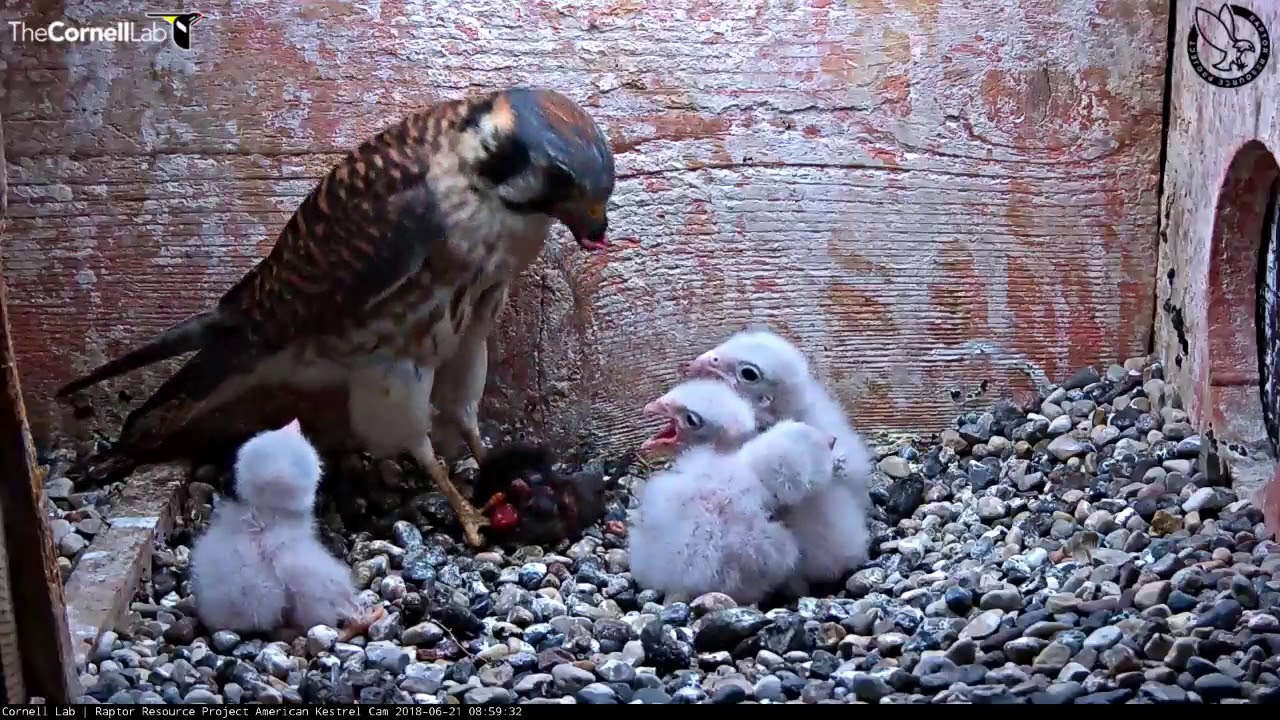This captivating image from the Cornell Lab showcases a smaller bird of prey, likely a falcon, within a wooden birdhouse. The birdhouse, intentionally designed with an entry hole, contains a bed of pebbles and rocks, creating a rocky ground for the birds. The adult falcon, characterized by its black head, brown feathers, and beige underbelly, is diligently feeding its four fluffy white chicks. These chicks, with their open pink mouths, are eagerly looking up at their mother as she tears pieces of meat, presumably from a recent catch, to nourish them. The tender moment captures the essence of maternal care and the natural behaviors of these majestic birds, emphasizing the powerful bond between the mother falcon and her offspring.